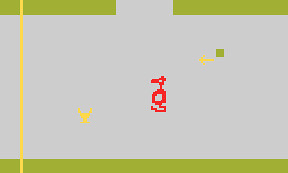The image depicts a retro video game screenshot from the Atari 2600 title "Adventure". The overall background is gray with green borders at the top and bottom, the top border being split into two with more gray in the middle, resembling an entrance or exit. On the left side, a thin yellow line runs vertically from the top to the bottom. The primary elements within the image include a red dragon, positioned as the central focal point, and two small yellow icons, one being the player character and the other an arrow, indicating direction. Near the top lies a green square behind the dragon. The image's pixelated and blocky nature further evidences its vintage origin.